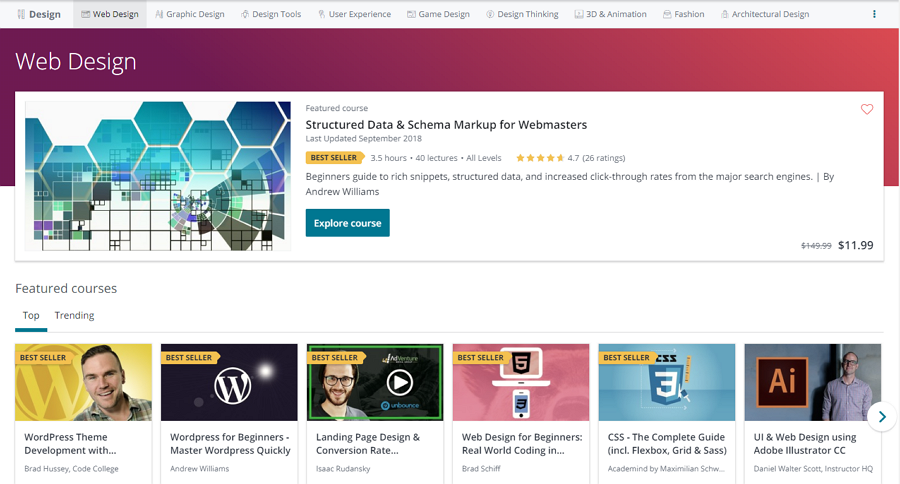Screenshot of an open website showcasing a variety of design-related courses. At the top, a white navigation bar spans across the width of the page, with options including "Design," "Web Design," "Graphic Design," "Design Tools," "User Experience," "Game Design," "Design Thinking," "3D and Animation," "Fashion," and "Architectural Design." On the right-hand side of the navigation bar, there are three blue dots indicating a pull-down context menu.

The main section of the screenshot features a vibrant banner with a gradient transitioning from purple to red, highlighting the "Web Design" category. Below the banner, a white square contains an image with blue hexagons and squares, promoting a featured course titled "Structured Data Scheme: Making Schema Markup for Webmasters." The course details include:
- Last updated: September 2018
- Bestseller tag with a yellow background and black text
- Duration: 3.5 hours
- 40 lectures
- Suitable for all levels

The course also displays a star rating of 4.7 stars from 26 reviews and is described as a "Beginner's Guide to Rich Snippets, Structured Data, and Increased Click-Through Rates" intended for the majority of major search engines. The instructor for this course is Andrew Williams.

A blue "Explore Course" button with white text invites users to learn more, and the price is prominently displayed as $11.99, reduced from the original $149.99.

Below this featured course section, the website showcases various "Top Trending" courses, all marked as bestsellers except for one. The courses listed include:
1. "WordPress Theme Development" by Brad Huxley, Code College.
2. "WordPress for Beginners: Master WordPress Quickly" by Andrew Williams.
3. "Landing Page Design and Conversion Rate Optimization" by Isac Radunski.
4. "Web Design for Beginners: Real Work Coding" (Instructor not fully visible).
5. "CSS: The Complete Guide Including Flexbox and Sass" by Maxine Academia.
6. "UI and Web Design using Adobe Illustrator CC" by Daniel Walter Scott, Instructor HQ.

An arrow icon at the bottom indicates that more courses are available to view beyond the current selection.